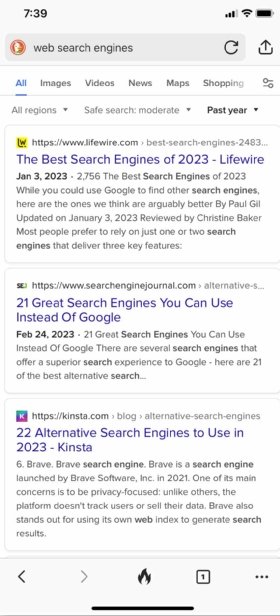The image depicts a screenshot of a web browser search engine results page. The status bar indicates a signal strength of 739, with full Wi-Fi and battery signals. The search query includes keywords such as "best search engines" and presents results spanning several categories shown in blue, including "All," "Images," "Videos," "News," "Maps," and "Shopping." Further filtering options are displayed in gray text, such as "All regions," "Safe Search," and "Moderated past year."

One highlighted search result is from the website www.livewire.com, titled "Best Search Engines 2023." This entry is dated January 3rd, 2023, and authored by Paula Gell, with an update on the same date. The article is reviewed by Chrissy McCormick and discusses how most people prefer using one or two primary search engines that offer comprehensive features and functionalities. Among the list of recommended alternatives, the text mentions notable ones identified by Chris Tyler Conn, who curated a list of 22 alternative search engines to use in 2023. The text emphasizes that these alternatives offer a potentially superior search experience compared to Google, suggesting users explore these options for varied and enhanced search capabilities.